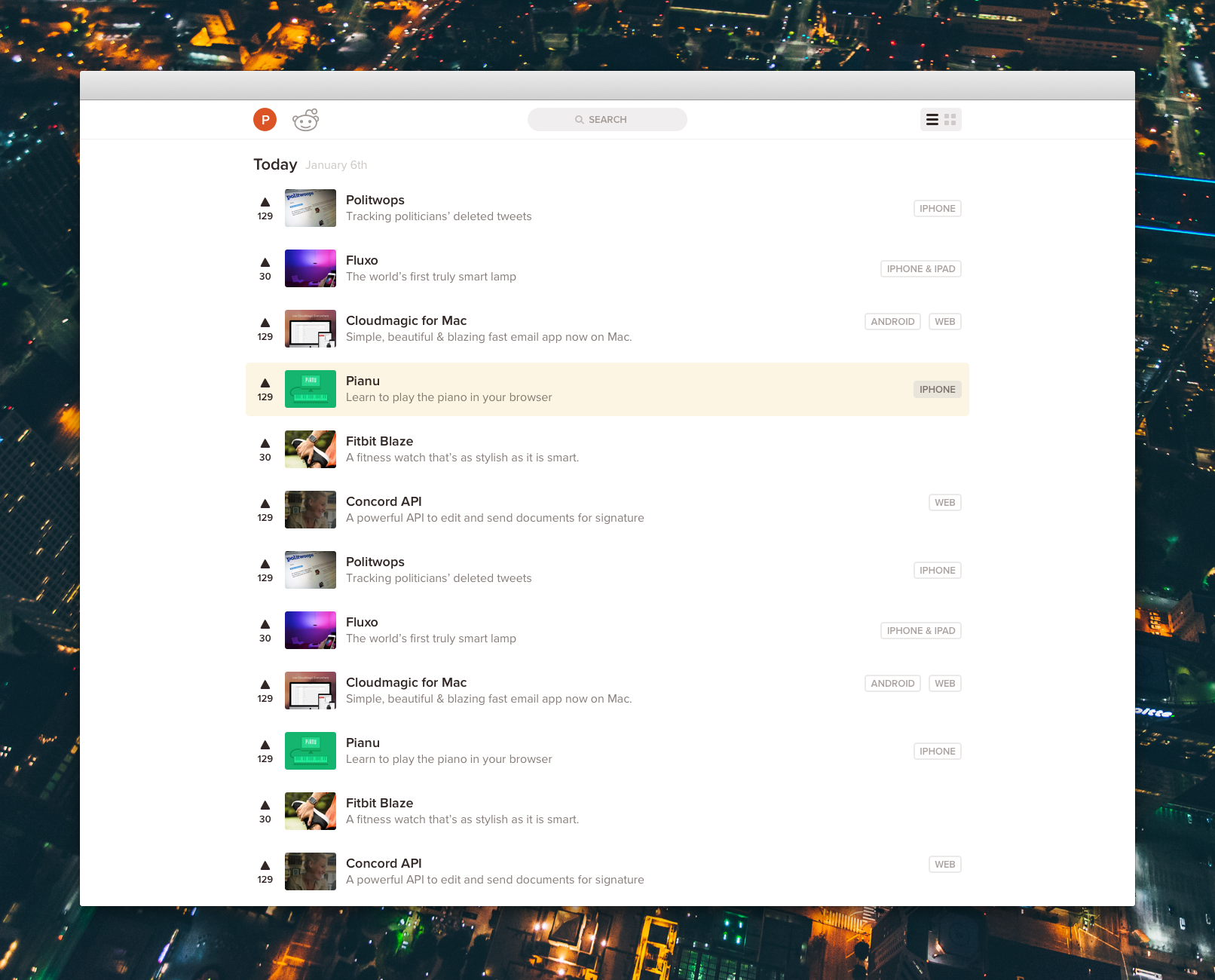The image shows a Reddit window open on a computer, likely a Mac given the design of the interface. The Reddit interface displays in an application window with a distinct white and grey theme common to macOS. The iconic Reddit mascot is visible in the top left corner, alongside a username starting with the letter 'P' and a central search bar. The date in the upper section is marked as January 6th, which holds historical significance. 

On the main screen, there are several posts visible, appearing to be a list of technology-related topics and products. Some notable posts include:

- "Poltywops: tracking politicians' deleted tweets" with 129 upvotes.
- "Fluxo, the world's first truly smart lamp" with 30 upvotes.
- "Cloud Magic for Mac: simple, beautiful, and blazing fast email app now on Mac" with 129 upvotes.
- "Planu, learn to play piano in your browser" with 129 upvotes.
- "Fitbit Blaze, a fitness watch that's as stylish as it is smart" with 30 upvotes.
- "Concord API: a powerful API to edit and send documents for signatures" with 129 upvotes.

Interestingly, the posts appear to repeat, making the feed seem more like a series of advertisements or sponsored content rather than a typical user-generated Reddit feed. Additionally, there are tags indicating compatibility with iPhone, Android, and web platforms next to some of the featured posts.